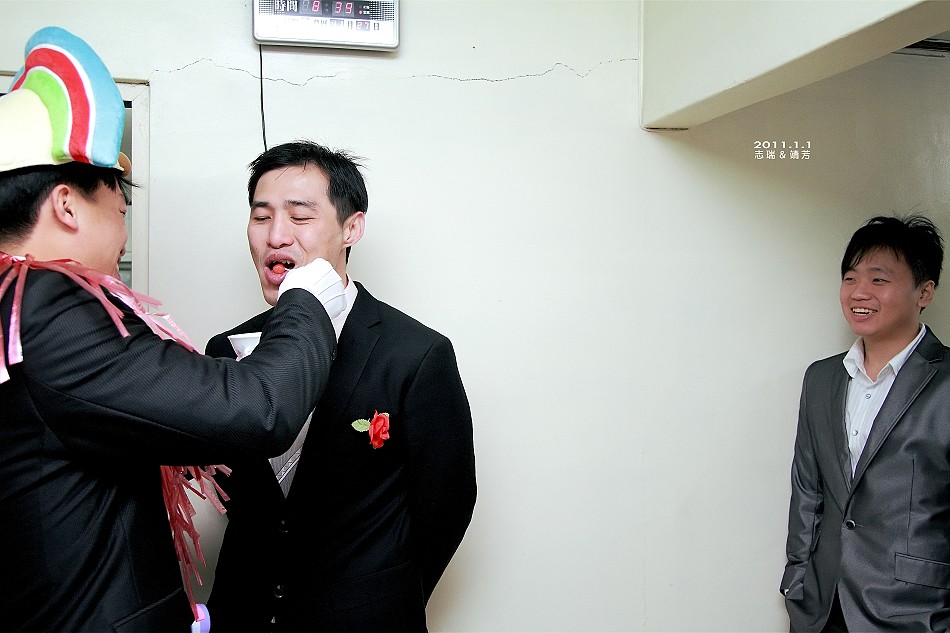The image, taken indoors in an older building characterized by white walls and a conspicuous crack running across the top, depicts a scene with three men in suits. Prominently, a man in a black suit with a red flower in his pocket stands beneath a clock that reads 8:39. This man, with black hair and a gray tie, has his mouth open as another man feeds him what appears to be a lollipop. The feeder is also wearing a suit, accented by white gloves, pink ribbons around his neck, and a blue, red, and green hat. To the right, another gentleman in a gray suit watches with a smile, seemingly amused by the activity. Above this spectator, the date '2011, 1, 1' and some Chinese text are visible, suggesting the setting is likely on January 1st, 2011, in a context of Chinese or Asian culture.